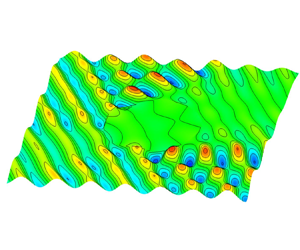The image displays an abstract, geometric design that is predominantly rectangular and wider than it is tall, featuring a visually striking assortment of vibrant, neon colors. The edges of the design are wavy, adding to its dynamic appearance. The left side is characterized by diagonal stripes in shades of blue, yellow, and green, creating a layered, textured effect. Interspersed throughout the pattern are clusters of small, colored circles in hues of yellow, blue, and red, contributing to a sense of organized complexity.

The design has a somewhat cartoonish quality, indicative of it being either digitally drawn or computer-generated rather than painted. The overall composition is reminiscent of a topographic map, with wavy lines and patterns that suggest elevation and depth. These lines, sometimes rendered in black, provide a sharp contrast to the neon color palette, which includes intense greens, blues, and yellows. The clean, precise lines and dots throughout give it an orderly yet dynamic appearance, making it an eye-catching piece of abstract art.